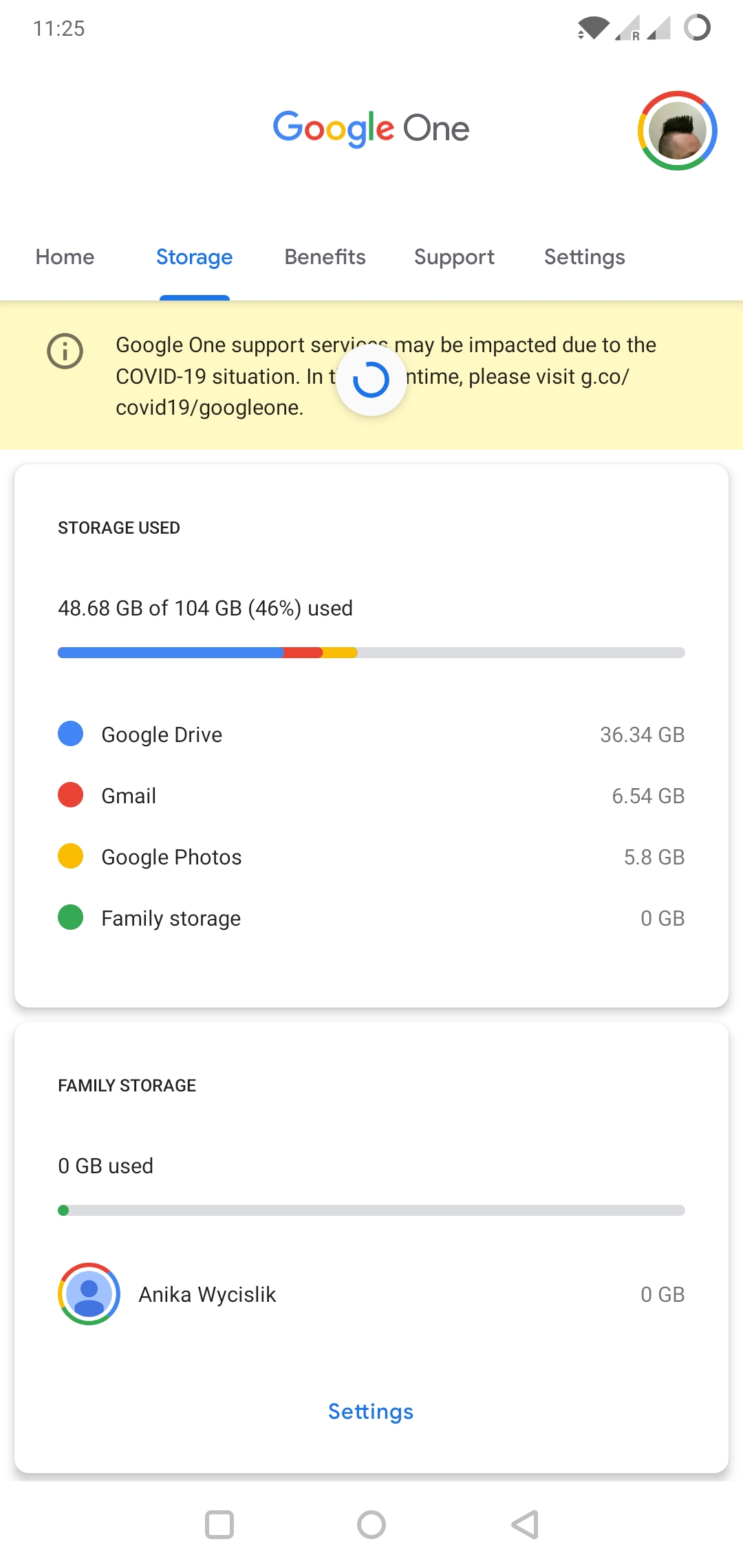This screenshot is taken from a phone and displays the Google One website. The background is primarily white, with a light tan-colored rectangle about an inch from the top. At the very top left, the time is shown as "1125" in black. On the right side, there is a small half-dark gray, half-light gray circle. Below it are two internet bars (one bar active), a fully-connected Wi-Fi icon, and a profile picture characterized by a gray background and a black mohawk at the top.

To the left of this profile picture, "Google One" is displayed in the classic Google colors. Further down, a horizontal menu includes options: "Home" in black, "Storage" in blue with an underline, followed by "Benefits," "Support," and "Settings" in black from left to right.

The tan-colored rectangle below features information about COVID, overlaid by a white circle containing a blue loading ring. Below that, a square with black lettering states "Storage used." This section provides a progress bar depicting storage usage: approximately one-third blue, followed by a small portion in red, yellow, and the remaining in gray. Underneath the bar are color dots (blue, red, yellow, green) from top to bottom, representing Google Drive, Gmail, Google Photos, and Family Storage, respectively. To the right of these dots, corresponding storage information is provided.

A little further down, another square labeled "Family Storage" shows "0 GB used," with an empty gray bar below. On the bottom of this square, there is another profile icon with the Google colors (red, blue, green, yellow) but without any internal details. Next to it, the name "Anaco Wycislik" appears, with "0 GB" indicated on the right side. Finally, below this section, there is a blue "Settings" label.